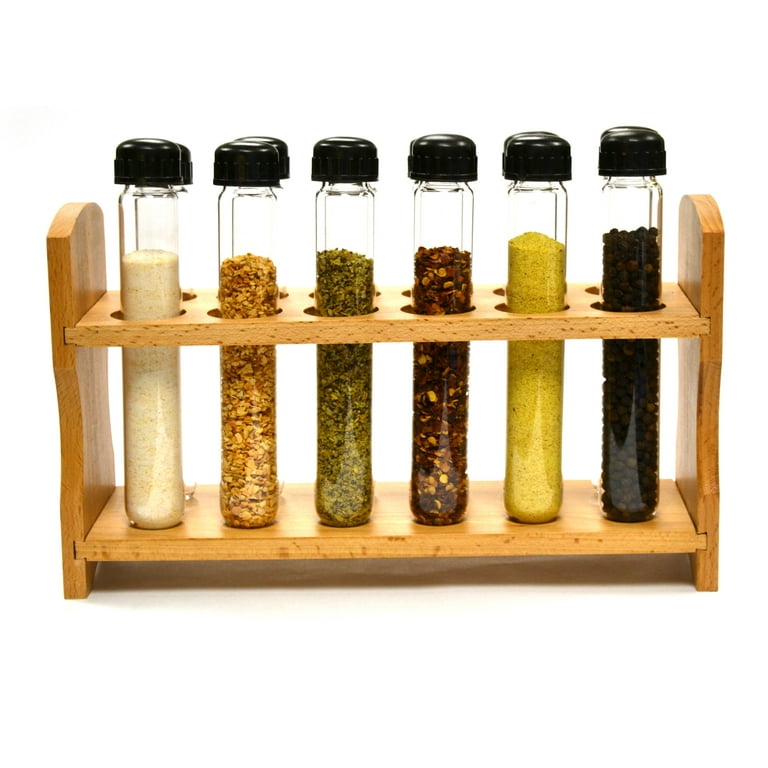This is a meticulously detailed and realistic photograph on a plain white background, showcasing a wooden tray that holds an array of long, slender glass test tubes, each with a black screw top. These twelve transparent tubes, arranged in two rows, primarily focus on the front row, which contains a variety of seasonings and spices. 

From left to right, the tubes are filled with the following materials:
1. A very white substance resembling either fine sand or finely flaked rice.
2. A brown, granola-like material.
3. A green herb that appears to be oregano or parsley.
4. A dark brown spice.
5. Yellow flakes that might be cornmeal.
6. Black peppercorns, recognizable by their round shape.

The second row behind these tubes mostly contains clear, empty bottles, emphasizing the utilization of the front row. The vivid colors of the seasonings allow for easy identification without labeling. The wooden tray provides an organized and aesthetic way to store these culinary ingredients, highlighting their textures and hues against the minimalist backdrop.